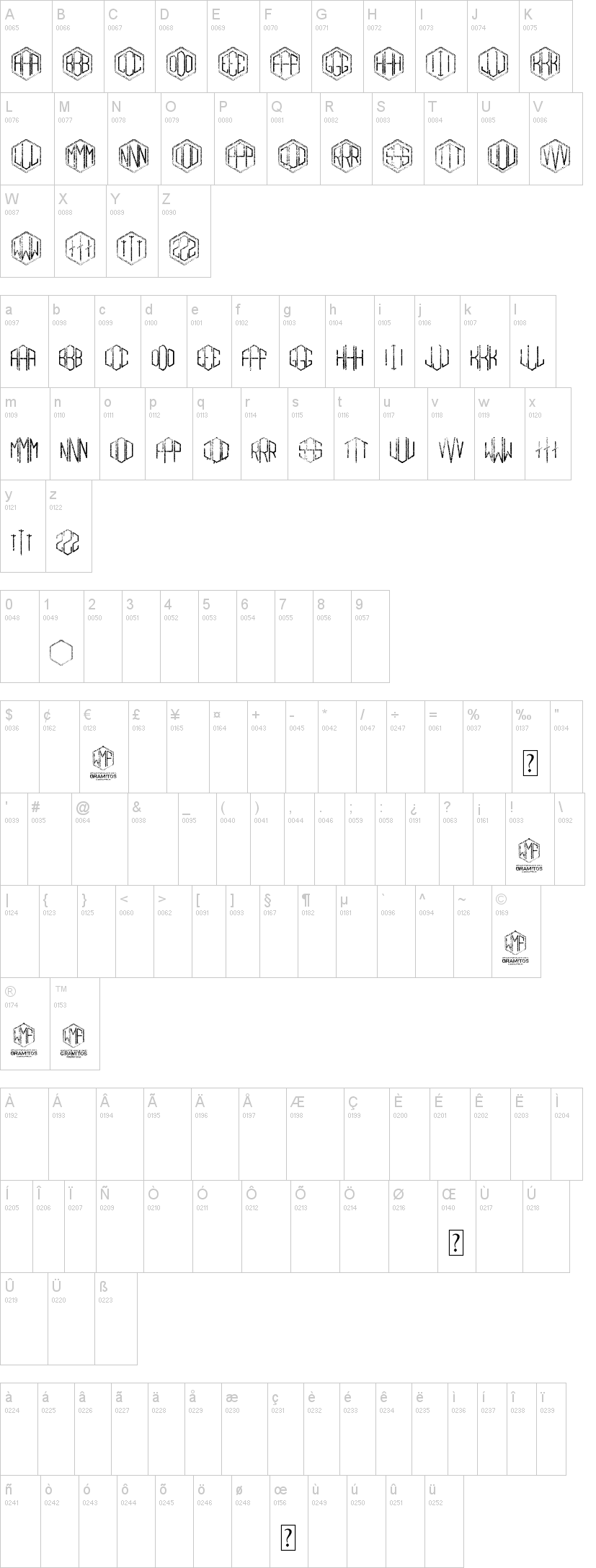This image is a detailed screenshot displaying a grid-like structure on a white background. The grid is arranged into multiple rows and columns, each containing individual boxes with letters and symbols. 

- The first row is labeled with uppercase letters from A to K, aligned at the top left corner of each box. Each box also contains a unique symbol, possibly resembling a hexagon with various internal line patterns.
- The second row continues with letters L through V, also positioned at the upper left corner of their respective boxes, each accompanied by different symbols as well.
- The third row is shorter and features the letters W, X, Y, and Z, with another run-through of the lowercase alphabet that starts from a and ends at k.
- Following this, rows of lowercase letters are depicted, starting from a to l, followed by m to x, and y to z.
- A numeric row is presented next, displaying digits from 0 to 9, with only the box under the digit 1 containing a symbol.
- There are additional rows where the letters and symbols become progressively less legible. The first of these additional rows includes three symbols: one in the third box, one in the penultimate box of the first sub-row, and one in the last position of the second sub-row.
- Subsequent rows have even more blurred and indecipherable letters or numbers. One of these rows features the letter 'A' repetitively, followed by a series of boxes each containing the letters C, E, and O. Symbols appear intermittently.
- Further down, the letters become more unclear, although it is mentioned that some parts include characters like 'B' and possibly 'O'.
- The final rows, though very blurry, include small, unreadable figures with a symbol in one of the boxes, fifth from the last, resembling a question mark.

This precise description captures the essence of the image, detailing the sequential order of letters, symbols, and their placements within rows and columns.